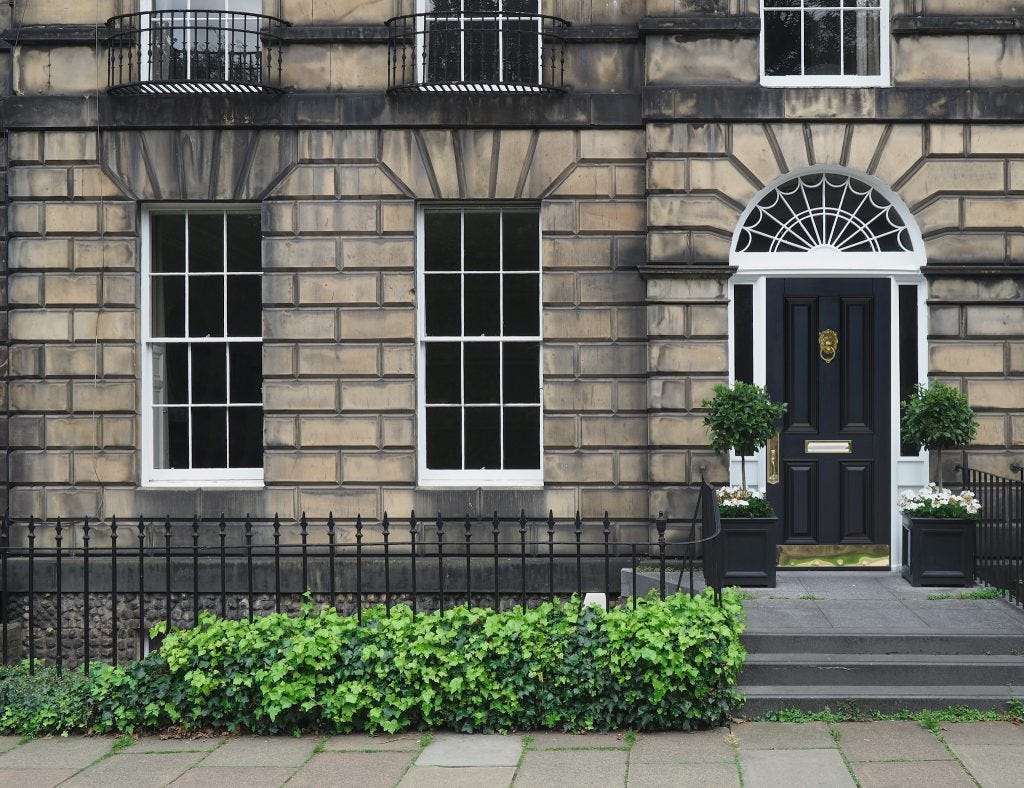This image appears to be a detailed illustration or highly realistic photo of a historic brownstone building with a tan and worn, stone-colored facade. The entrance, located on the right side, features a deep black door adorned with gold hardware, including a lion’s head knocker, mail slot, and door handle. The door is framed by white trim and flanked by two white-framed vertical windows. Above the door is a half-circle window with a decorative spiderweb design in white.

To the left of the door, there are two white-trimmed windows with multiple panels and darkened glass that prevents seeing the interior. The base of the building has brown to gray stone slabs, slightly worn, with patches of grass and weeds poking through the gaps. In front of the stone slabs is a bright green hedge, backed by a black iron palisade fence that runs along the property on the left side, helping to prevent falls to the basement level. Along the sidewalk, which is composed of square stone tiles with occasional weeds growing in between, there are gray steps that lead directly up to the front door.

Both sides of the entrance porch are flanked by black planter boxes containing decorative trees and white flowers, adding to the building’s welcoming aesthetic. The exterior walls of the building appear to be made of old, sooty brown bricks, contributing to its historic charm. The overall scene suggests an elegant, lived-in property with a mixture of natural and architectural details that enhance its character.